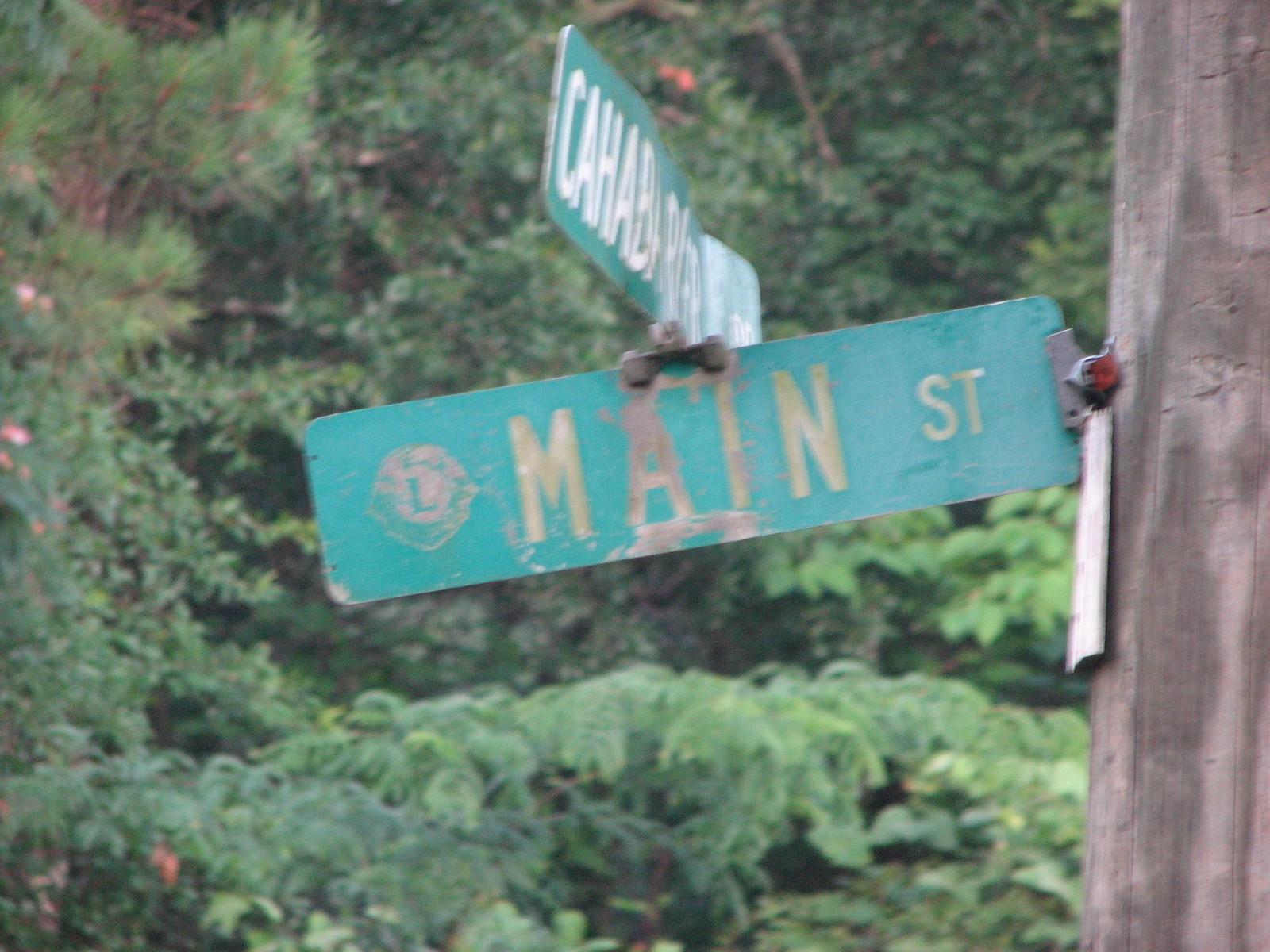The photograph captures a somewhat weathered street sign affixed to a wooden lamppost on the right edge of the frame. Dominantly featuring "Main Street" in white, albeit faded, lettering against a green background, the sign appears tilted and aged, with hints of moss or algae. Above it, a newer, crisper green sign with white letters reads "CAHABA," though not fully legible. The wooden pole shows varying shades of brown but remains in good condition. The scene is set against a vibrant backdrop of lush greenery, with both needle-bearing and deciduous trees. Rich foliage and diverse textures, from lighter leafy greens to brownish-orange branches, create a vivid, natural environment surrounding the pole and signs.